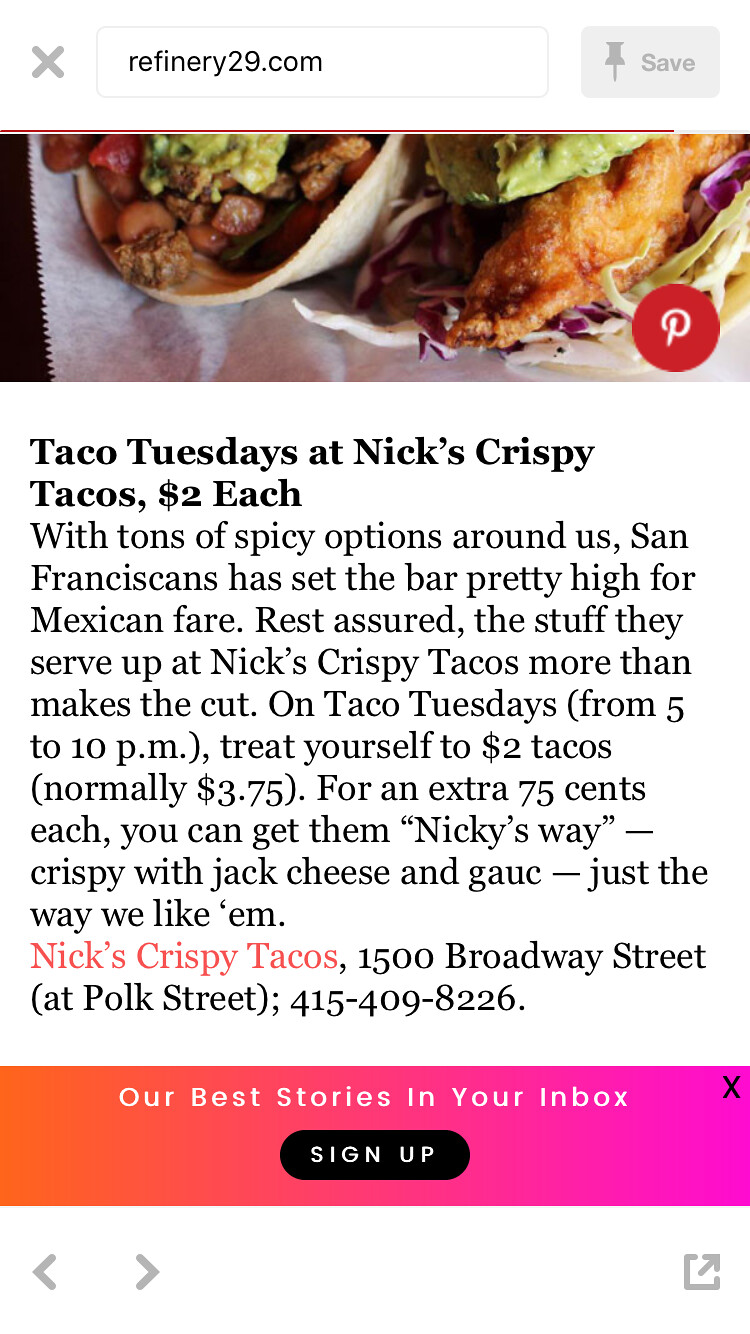This image appears to be a colorful phone screenshot from the website Refinery29.com, showcasing an advertisement for Taco Tuesdays at Nick's Crispy Tacos in San Francisco. At the very top, there's a web address bar, with save and close buttons. In the lower right corner, the Pinterest logo hints at the source. The vibrant photograph, presumably of chicken tacos, sits prominently at the top. The bold black text announces, "Taco Tuesdays at Nick's Crispy Tacos, $2 each," with the promotional hours of 5-10 p.m. Normally priced at $3.75, these tacos can also be ordered Nicky's Way for an extra $0.75, adding jack cheese and guacamole for a crispy twist. The description proudly highlights San Francisco's high standards for Mexican fare and assures that Nick's Crispy Tacos meets those expectations. The restaurant is located at 1500 Broadway Street at Polk Street, with a contact number of 415-409-8226. The bottom of the page features a sign-up prompt for Refinery29's best stories, accompanied by a color gradient banner ranging from orange, pink to purplish hues, with navigation arrows on either end.